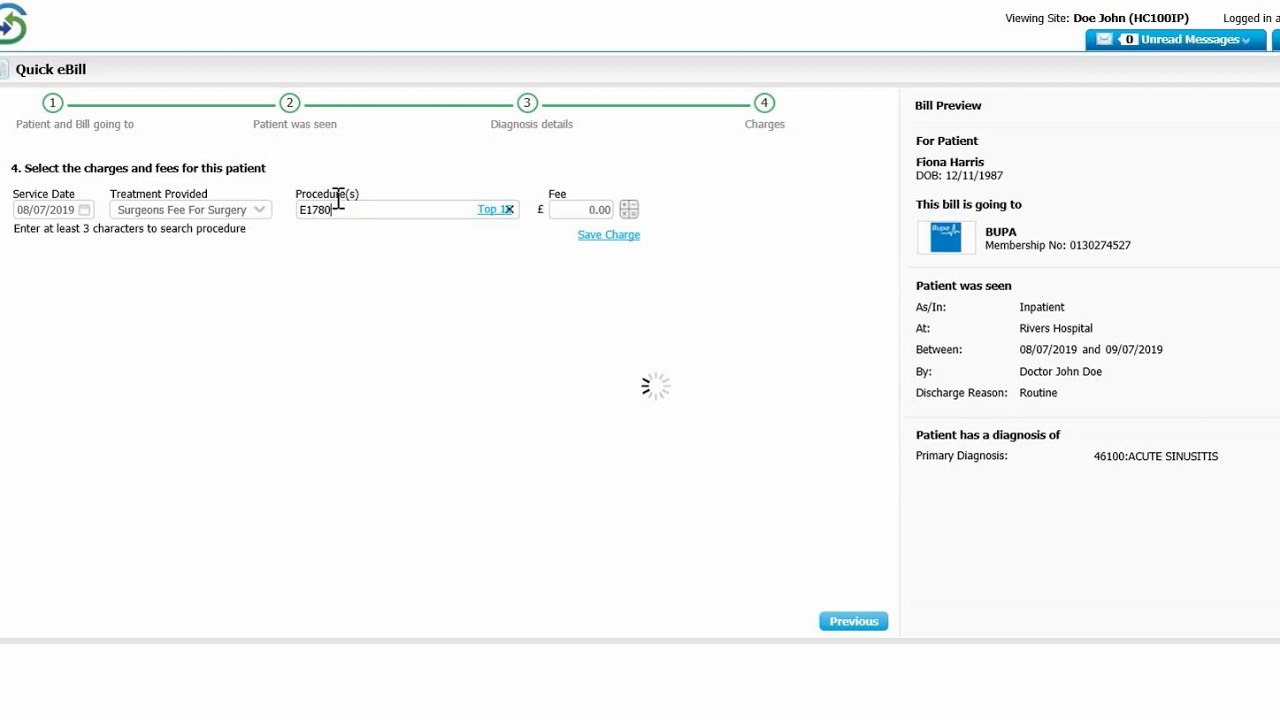This is a screenshot taken from an unidentified website. 

At the top, there is a white banner adorned with a stylized icon featuring blue and green curving arrows arranged in an S formation. On the upper right of the banner, the navigation text reads:
- "Viewing Site, Doe, DOE, John, HC 100 IP"
- "Zero unread messages"
- "Click E-Bill"

Below this, the sections are outlined numerically as follows:
1. "Patient and bill going to"
2. "Patient was seen"
3. "Diagnosis details"
4. "Charges"

In the "Charges" section, there are detailed instructions and fields, stating:
- "Select the charges and fees for this patient"
- "Service date: 8-7-2019"
- "Treatment provided: Surgeon’s fee for surgery"
- "Procedure: E-1780"
- "Fee: £0.00"
- "Enter at least three characters to search procedure"
- "Save change, save charge"

To the right, there is additional information under the heading:
- "Bill Preview for Patient Fiona Harris"
- "DOB: 12-11-1987"

The billing details specify:
- "This bill is going to: BUPA"
- "Membership number: 0130274527"
- "Patient was seen as an inpatient at Rivers Hospital between 8-7-2019 and 9-7-2019 by Dr. John Doe"
- "Discharge reason: Routine"
- "Patient has a diagnosis of: Primary diagnosis 46-100 acute sinusitis"

At the bottom, there is a blue rectangular button labeled "Previous".